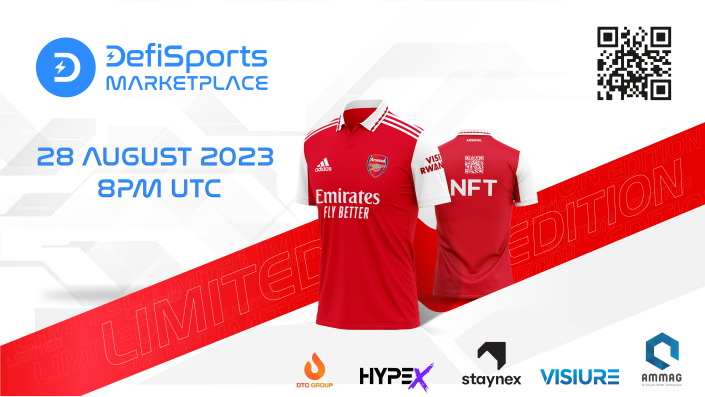The advertisement features two red athletic jerseys with white sleeves and stand-up collars, prominently displayed against a white background. A striking red ribbon runs diagonally across the center of the image, bearing the words "Limited Edition." The foreground jersey, angled to the left, showcases the white decal "Emirates Fly Better" on the chest, accompanied by the Adidas emblem and additional patches on the top left, right, and side sleeve. The jersey in the back faces the viewer, also displaying "Emirates Fly Better" prominently.

In the top left corner, the banner bears the blue logo of "Defy Sports Marketplace," along with the event details: "28 August 2023, 8 p.m. UTC." The top right corner includes a black and white QR code for further information. The bottom of the poster features sponsor logos, including Hypex and Staynex. The combination of photographic realism and graphic design elements creates an eye-catching and detailed visual.